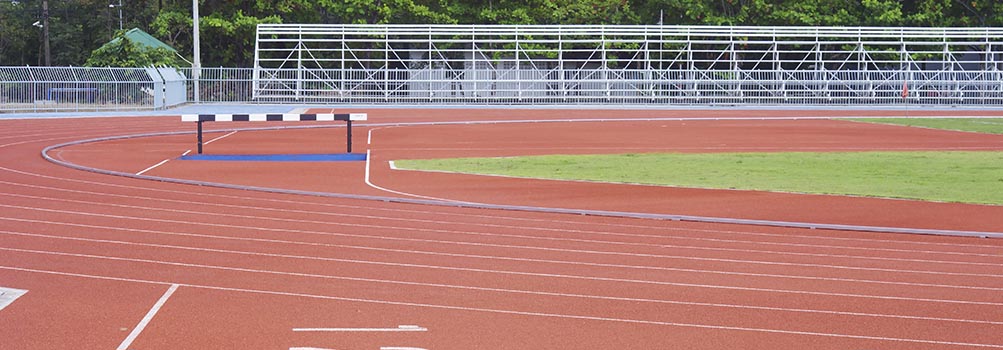This image captures a vibrant high school athletics stadium on an overcast gray day, emphasizing both the track and the surrounding scenery. The track, consisting of at least eight lanes, features a reddish-pink surface with crisp white lines delineating each lane. Scattered along the track are hurdles, one of which has a blue base topped with a black and white bar, indicating preparations for running and hurdle events. Encircling the track is a lush, green field used for various track and field sports. In the background, a row of metal bleachers awaits spectators, positioned in front of a metal fence. Beyond the confines of the track, a dense line of plush, full trees suggests either spring or fall, adding a natural, serene backdrop to the athletic setup. A small building can also be seen peeking through the trees, completing the scene with minimal sun and barely any shadows.